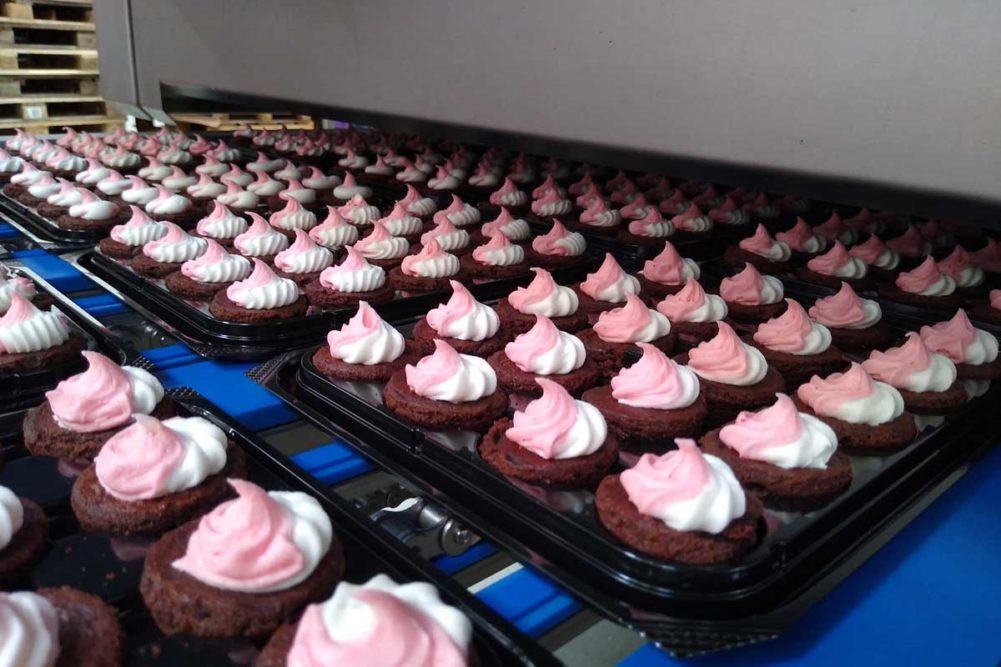In this color photograph, we see a close-up view of an assembly line featuring a remarkable display of uniform chocolate cupcakes. Each dark brown cupcake is precisely topped with a two-tone meringue-style frosting: a base of white with a pink swirl at the tip. The cupcakes are neatly arranged on black plastic trays, and there are about nine trays visible, stacked on a blue rack beneath them. Each tray supports several rows of these desserts, creating an organized and visually appealing alignment. The front rows of cupcakes are in sharp focus, while the back rows gradually blur out, highlighting the orderly craftsmanship.